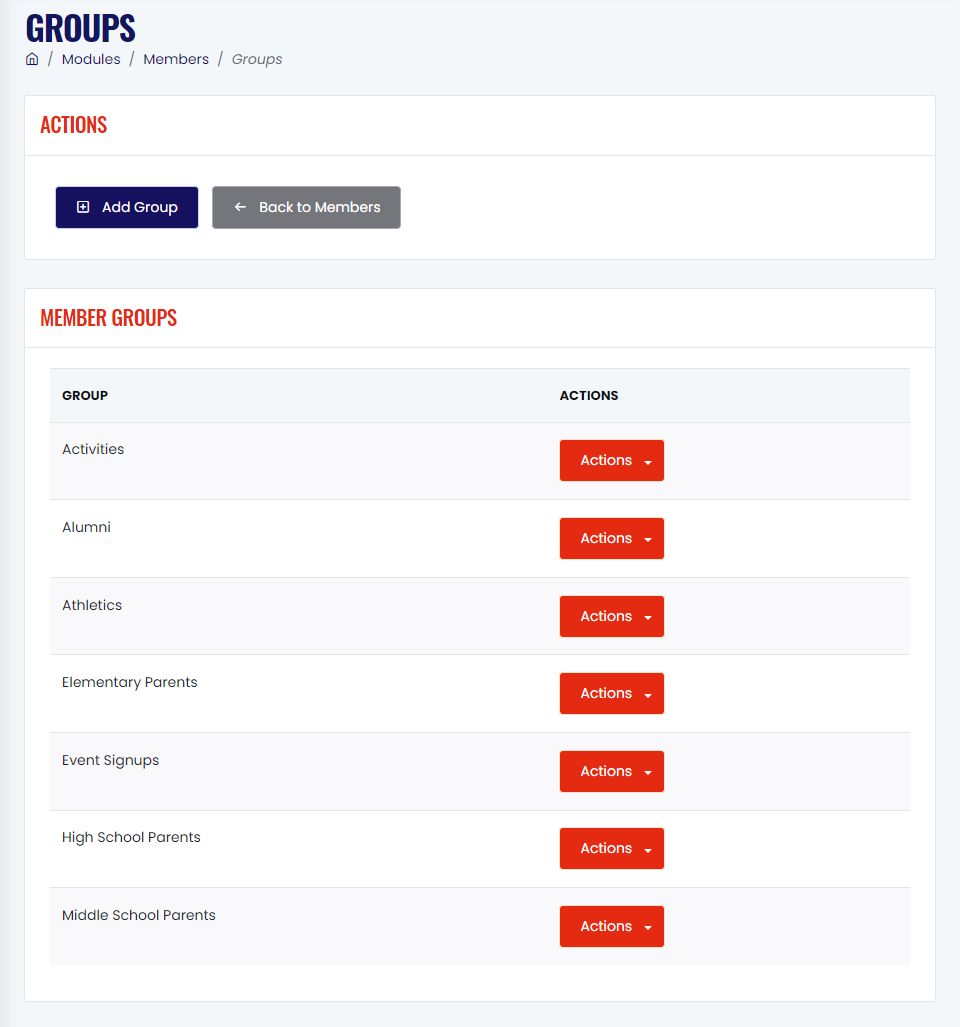This screenshot captures the layout of a website page. The background features a light gray top border, transitioning to a broader space with a dark blue font. At the very top, the title "Groups" is prominently displayed. Just below this title, there's a breadcrumb navigation path: a house-shaped icon followed by forward slashes, indicating "Modules / Members / Groups."

Beneath this navigation path, a white rectangular section features a red font header labeled "Actions." Below this section, another white rectangle contains two distinct buttons: a blue button labeled "Add Group" and a gray button labeled "Back to Members."

Further down, a detailed list is presented, organized into columns. The header in red font reads "Members Groups." The columns are labeled "Group" on the left side and "Actions" on the right side. Under the "Group" column, several categories are listed: "Activities," "Alumni," "Athletics," "Elementary Parents," "Event Sign-Ups," "High School Parents," and "Middle School Parents." Corresponding to each group name under the "Actions" column is a small red rectangle. Each rectangle includes the white text "Actions," accompanied by a drop-down menu icon that users can click next to each group name. The list alternates in background color between gray and white for each group name, providing a clean and organized appearance.